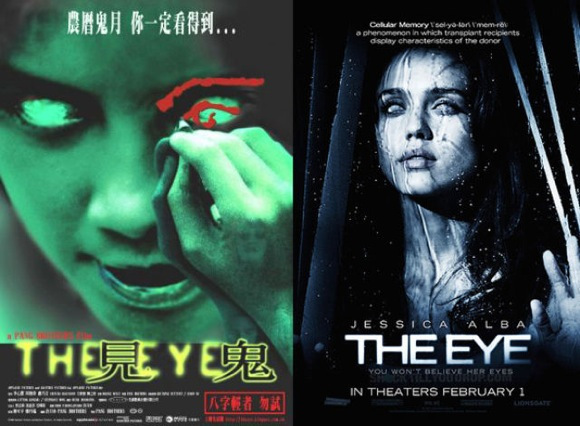In the image, there are two movie theater posters displayed side by side. The poster on the left is primarily in Japanese, featuring white text at the top and yellow text at the bottom. Dominating the image is a person with green skin, looking quite scary as someone is drawing on their eyebrow and eyeball with a red pen. The poster exudes a chilling atmosphere with its green and black color scheme. The poster on the right showcases a black and white image of Jessica Alba with her eyes whitened as if she is staring out a window with rain and curtains. The text on this poster reads, "Jessica Alba, The Eye, You Won't Believe Her Eyes," and it specifies the release date as "In Theaters February 1st." Both posters convey a sense of eerie intrigue, enhancing the overall unsettling vibe of the image.